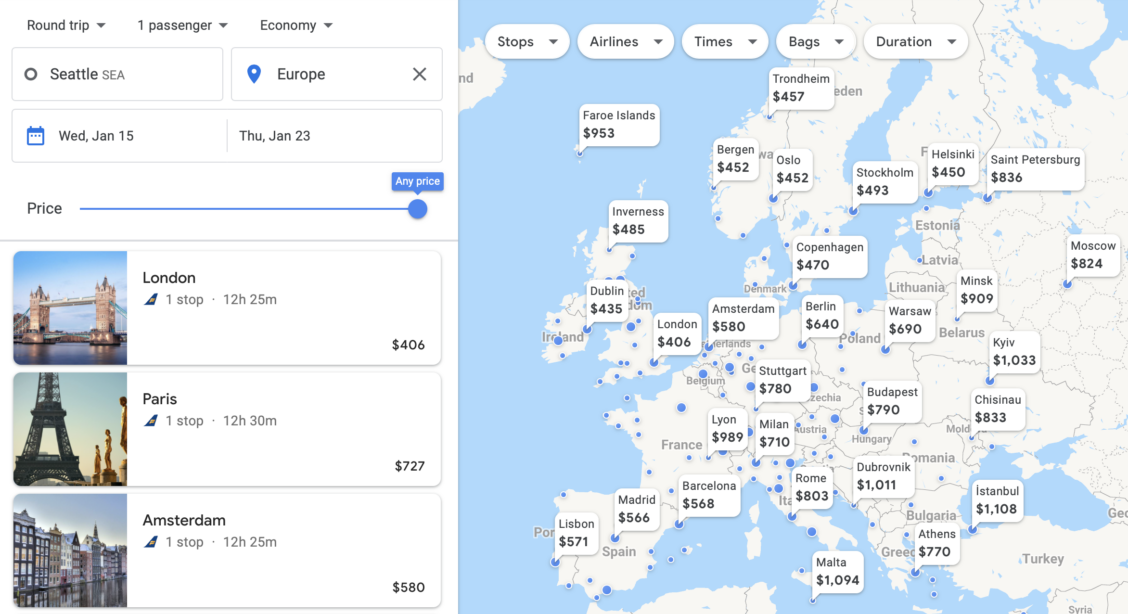The image features a detailed map of Europe on the right, showcasing flight prices to various major cities. At the top of the image are capsule-shaped buttons in white with drop-down arrows, each labeled in black font with options such as "stops," "airlines," "times," "bags," and "duration." Speech bubbles next to the cities indicate flight prices, such as Stuttgart at $780, Milan at $710, Lyon at $989, and Dublin at $435.

On the left-hand panel, which is white, several options are listed: "round-trip," "one passenger," and "economy," each with respective drop-down menus. The departure and arrival locations are set from Seattle (SEA) to Europe, marked with a blue location icon and an X. Travel dates are specified as Wednesday, January 15th to Thursday, January 23rd. A price range line shows the selection is set to "any price," indicated by a blue circle at the top of the line.

Additional details include images of iconic landmarks: London’s Tower Bridge against a blue sky, Paris’ Eiffel Tower at sunrise, and Amsterdam's canal-side buildings. Specific flight information is also provided, such as a flight to London being a one-stop journey lasting 12 hours and 25 minutes, priced at $406. A flight to Paris is a one-stop trip taking 12 hours and 30 minutes, costing $727. Finally, Amsterdam is reachable via a one-stop flight of 12 hours and 25 minutes, priced at $580.